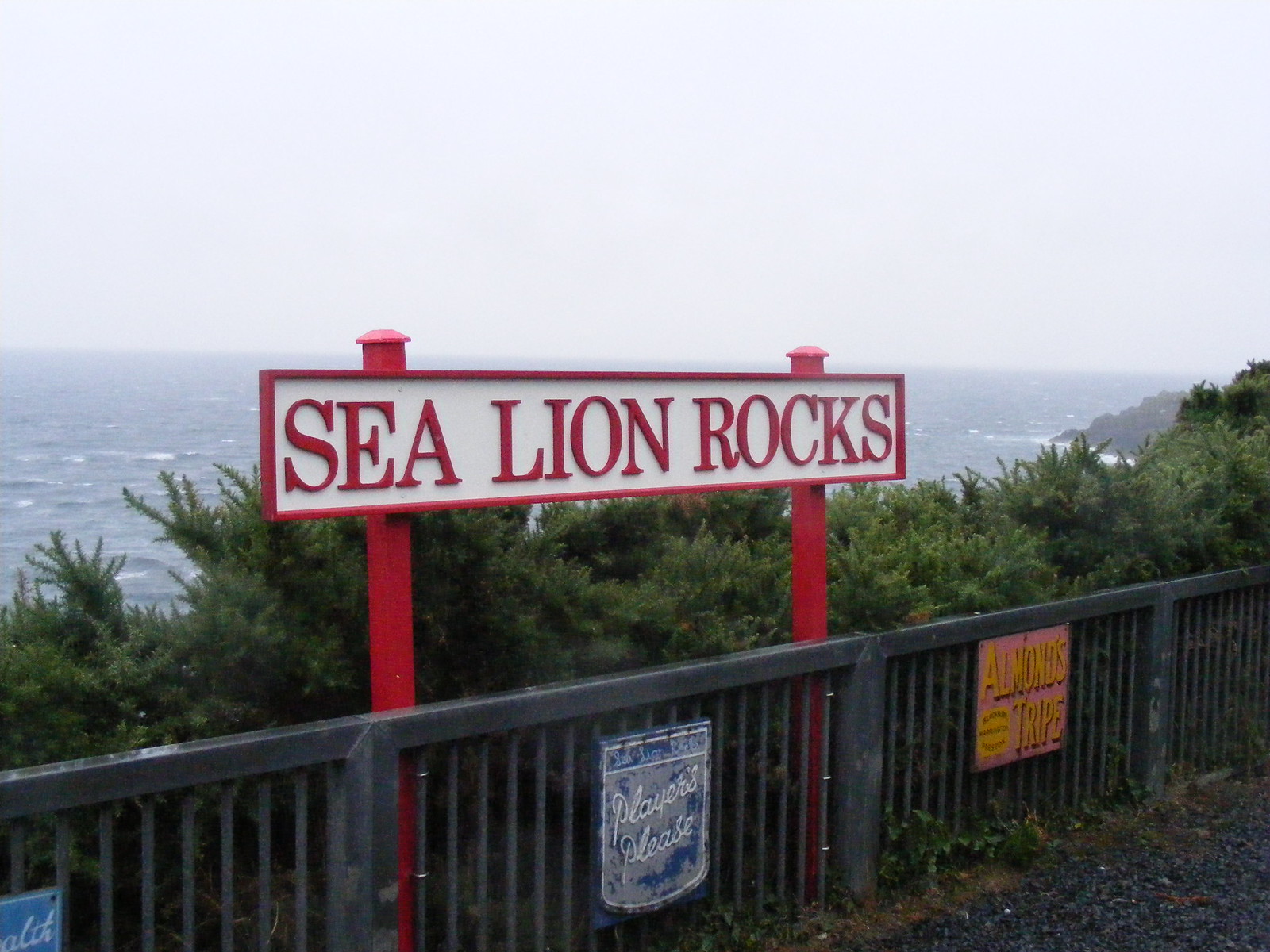The photograph captures a scenic coastline view framed by a sturdy black metal fence with vertical bars and scattered black gravel at its base, likely damp from a recent rain. Dominating the scene is a large horizontal rectangular sign, prominently positioned on two bright red posts about five to six feet high. The white background of the sign is accentuated by a red border matching the posts, with bold red letters spelling out "Sea Lion Rocks." Surrounding the sign, evergreen shrubs typical of coastal vegetation provide a lush backdrop.

Several smaller signs are attached to the fence itself, displaying messages like "Almond Stripe" and "Players Please," though one sign remains partially obscured. Beyond the fence and shrubbery, a rugged cliff edge drops off into the expansive, choppy waters of the sea, stretching out to a flat horizon beneath an overcast sky. Off to the right, the rocky coast gently tapers into the water, adding a dynamic element to the scene. The misty fog in the distance and whitecaps on the waves contribute to the image's dramatic, untouched quality, emphasizing the wild beauty of the landscape.